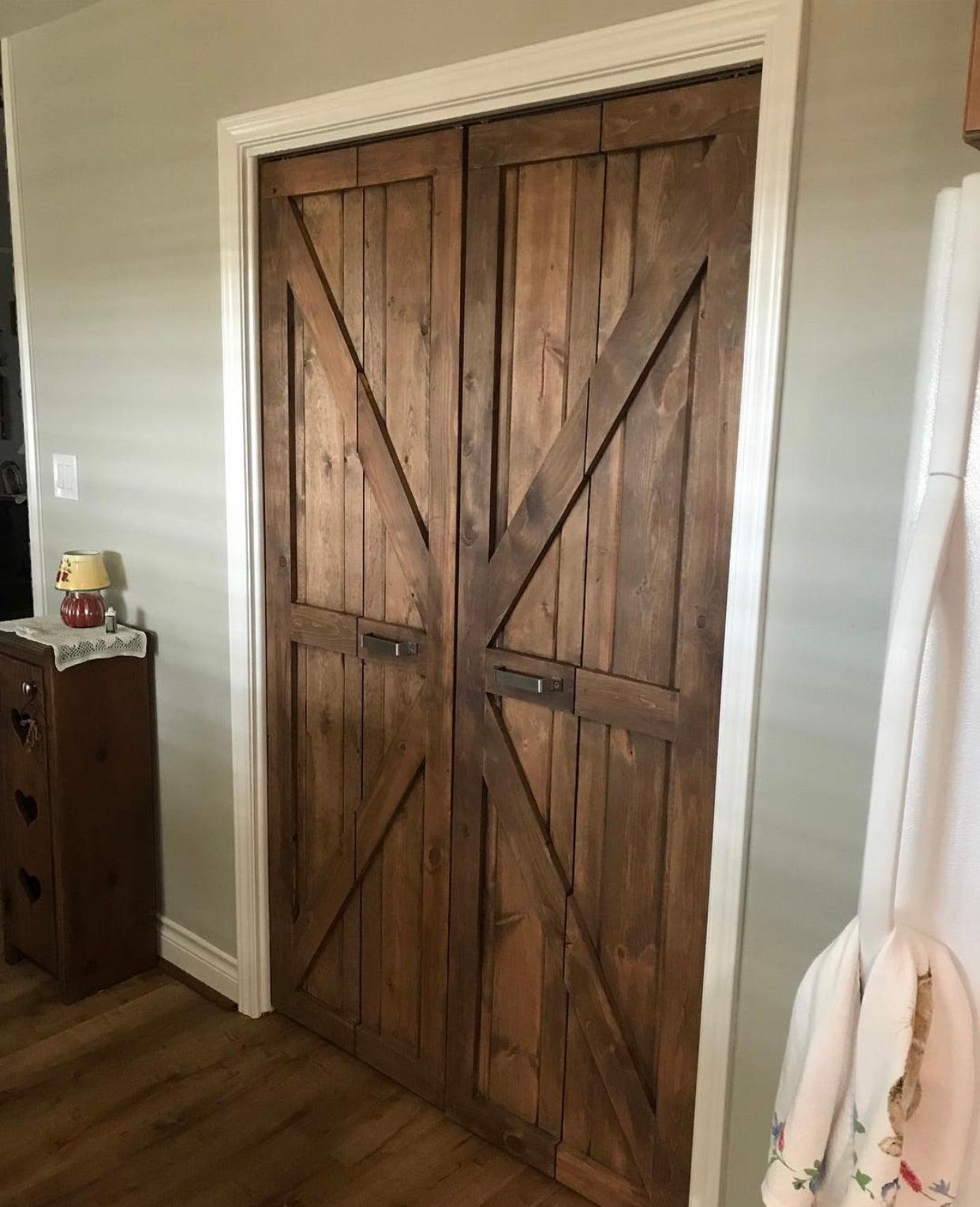This photograph, taken from the inside of a farmhouse-style home, prominently features a pair of rustic barn-style doors at its center. The vertically oriented image allows a full view of the doors, which are made of dark wood with varying tones. Each door is divided into four panels by a prominent "X" design formed by cross two-by-fours. These doors are double and appear to swing open, with two metal handles—silvery gold in color—positioned horizontally in the middle of each door. The doors are framed by white trim and baseboards against walls painted in a grayish-beige color, possibly with an olive undertone.

To the right of the doors is a partial view of a white refrigerator, identifiable by its vertical handle and a dish towel hanging at the bottom. Below the light switch on the left, there's a small brown side table with drawers featuring heart-shaped cutouts, topped with a white tablecloth. The table also holds a tiny, white and yellow lamp. The overall aesthetic blends modern touches with rustic farmhouse charm, creating a warm, updated look.